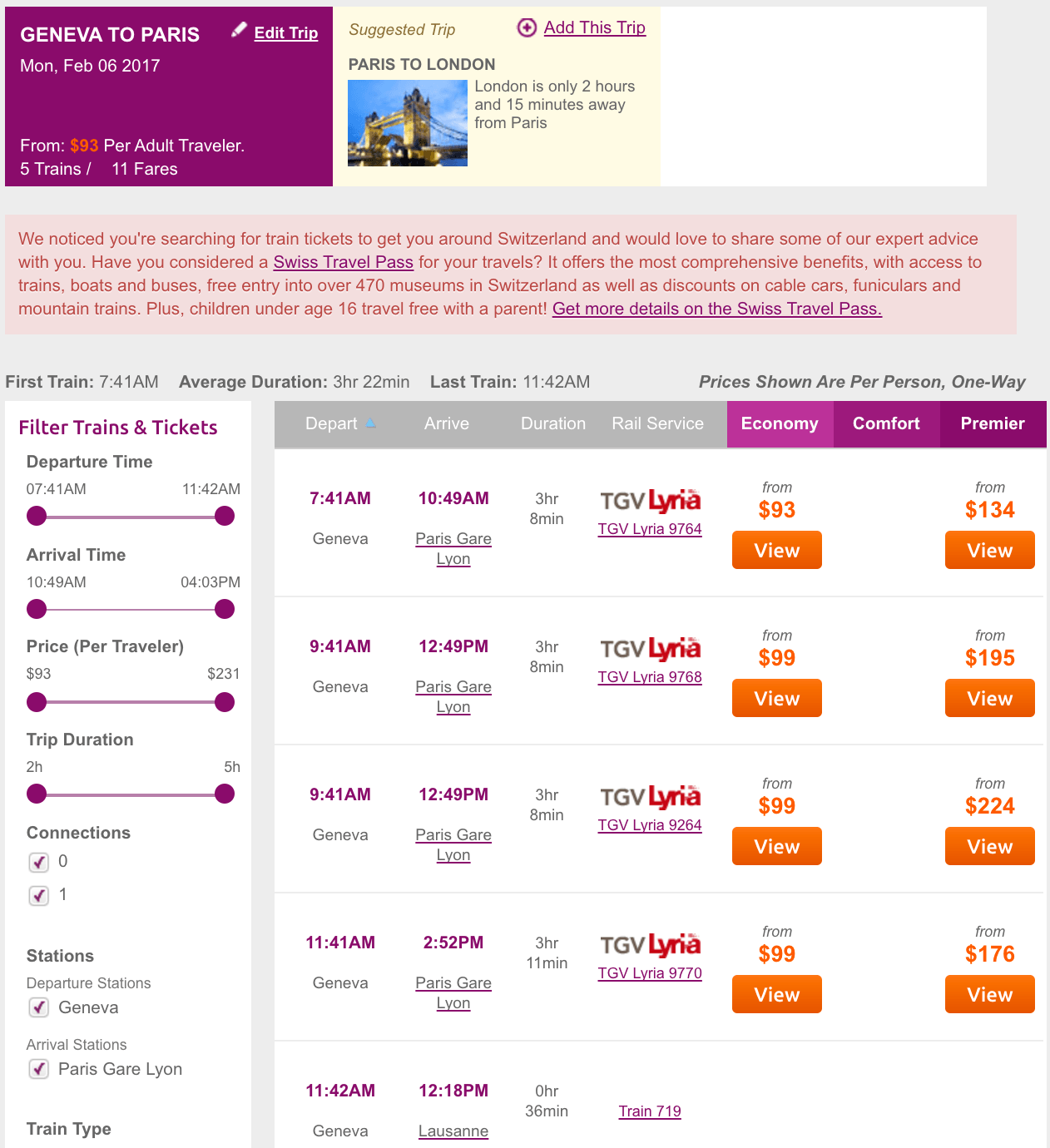The image depicts a flight booking website. The user is searching for a trip from Geneva to Paris on Monday, February 6, 2017. This information is displayed in a purplish-colored box located at the top left corner, along with the cost per adult ticket starting at $93. The search results indicate there are 5 available trains and 11 fares.

To the right, a yellow box suggests an additional trip option from Paris to London, noting that the journey takes only 2 hours and 15 minutes.

Below, a red-highlighted box notifies the user that they are searching for train tickets around Switzerland and offers expert advice, including a recommendation to consider a Swiss Travel Pass for their journey. 

The main section of the page lists available flights, including times: 7:41 a.m., 9:41 a.m., 11:41 a.m., and 11:42 a.m. All these flights are operated by TGV Lyria Lina with varying prices.